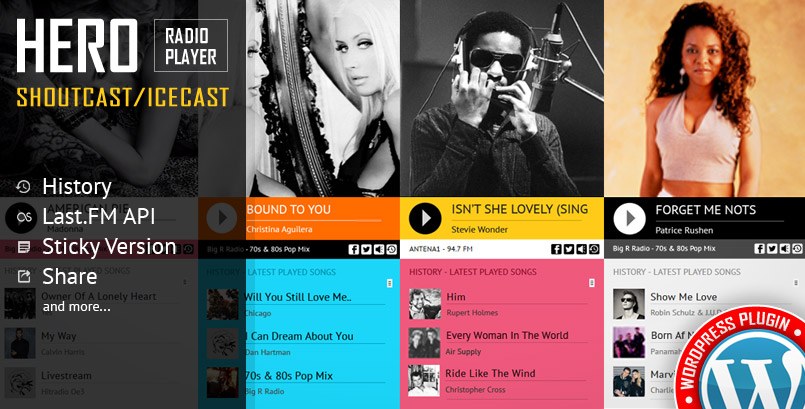In this image, we see a detailed screenshot featuring three distinct photographs of artists. Starting from the upper right corner and moving left, we first encounter an image accompanied by the text "Forget Me Nots" by Patrice Rushen. This photo showcases Patrice, a young woman with black curly hair, wearing a cream-colored halter top. Beneath the play button, it reads "Big R Radio, 70s and 80s pop mix."

To the left, there is an image of a young Stevie Wonder. In this vivid shot, Stevie is seated in front of a microphone, wearing earphones and his iconic black sunglasses. His hands are raised to his face, holding a harmonica. The caption beneath this image reads “Isn’t She Lovely, Stevie Wonder.”

Adjacent to Stevie Wonder’s image, on the far left, is a black-and-white photo of Christina Aguilera. The caption reads "Bound to You, Christina Aguilera". In this evocative shot, Christina is standing in front of a mirror, gazing thoughtfully at her reflection.

In the upper left corner, aside from these three chosen images, white text reads "Hero Radio Player". Beneath this, in yellow text, it says "Shoutcast Icecast."